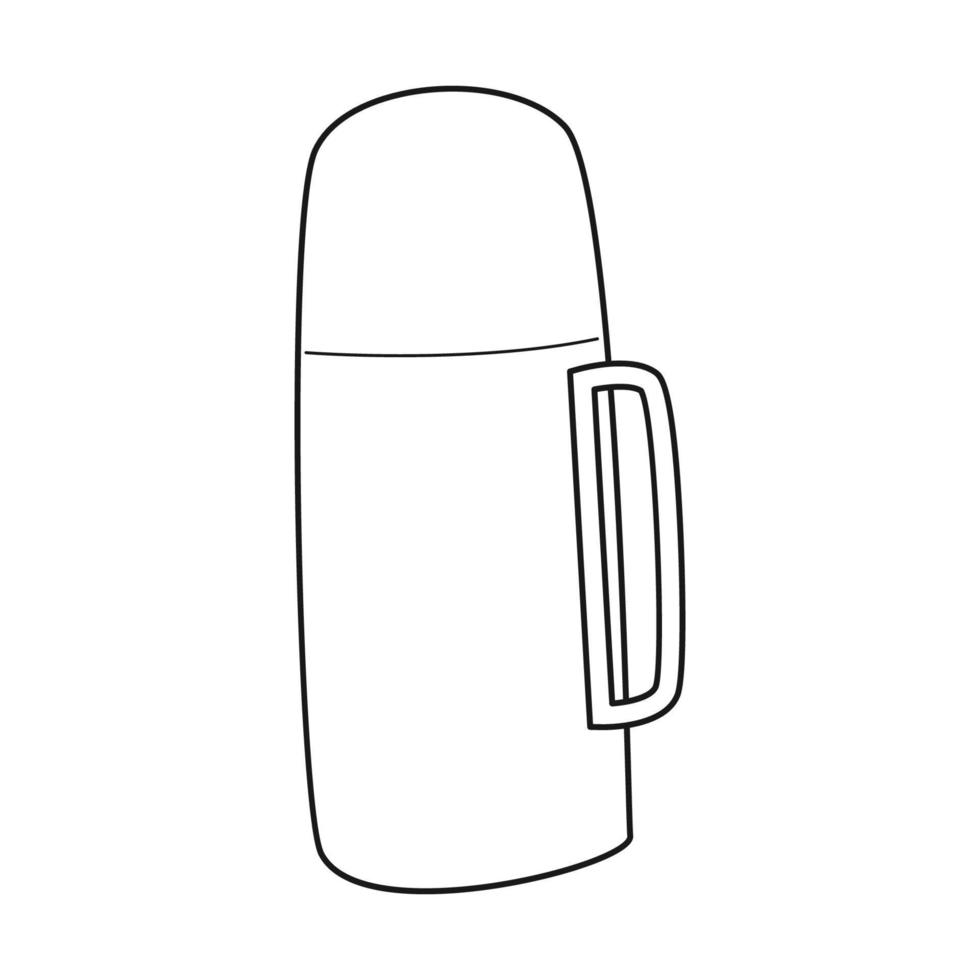This hand-drawn, black and white line illustration depicts a cylindrical jug or thermos, prominently featuring a side handle shaped like a capital letter "D". The object, centered against a solid white background with no text or border, appears to be outlined in what resembles black marker. A distinct horizontal line near the upper half, but not at the topmost point, indicates where a screw-on lid might be. The handle, also outlined in black, is attached to the right side of the thermos, enhancing its usability. The simplicity of the black lines against the white background highlights the thermos as the sole focus of this minimalist drawing, showcasing the artist's intent to emphasize the form and function of the object.